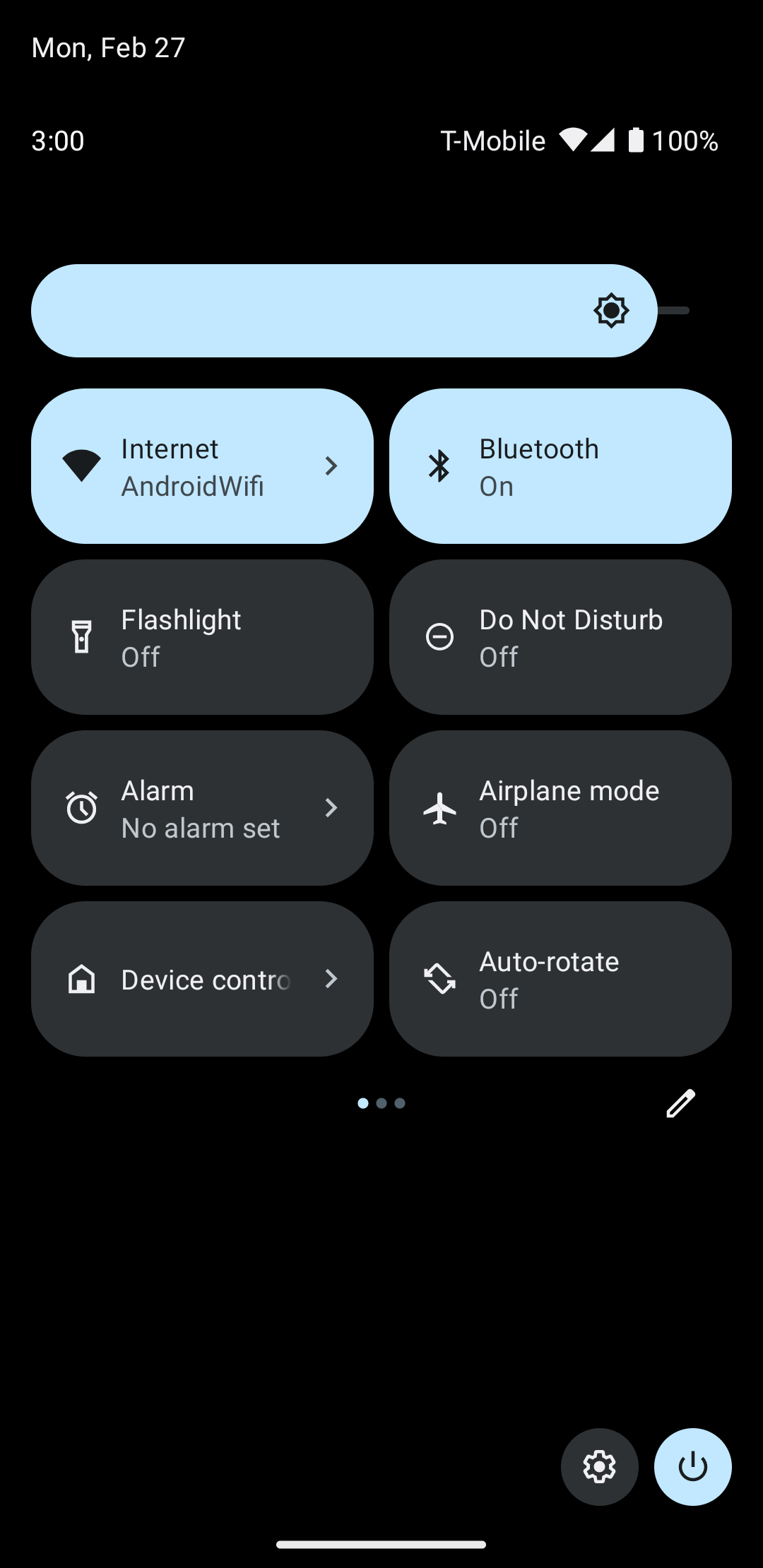In this image set against a solid black background, the focus is on a smartphone screenshot. In the upper left corner, in light gray text, is the date "Monday, February 27th," with the time displayed just below it as "3:00 PM." Adjacent to the time, "T-Mobile" is indicated as the service provider, with the Wi-Fi icon illuminated, and the battery level shown at 100%.

Directly beneath these indicators is a pale blue search box, followed by a series of control and status indicators. On the left, a rectangle outlines categories labeled as "Internet, Android, Wi-Fi." To its right, the Bluetooth status is marked as "on."

Below this section, various control boxes are listed: "Flashlight" is turned off, "Do Not Disturb" mode is off, no alarms are set, "Airplane mode" is off, and both "Device Control" and "Auto Rotate" are off. In the lower right corner of the image, the settings icon is prominently displayed, inviting further customization.